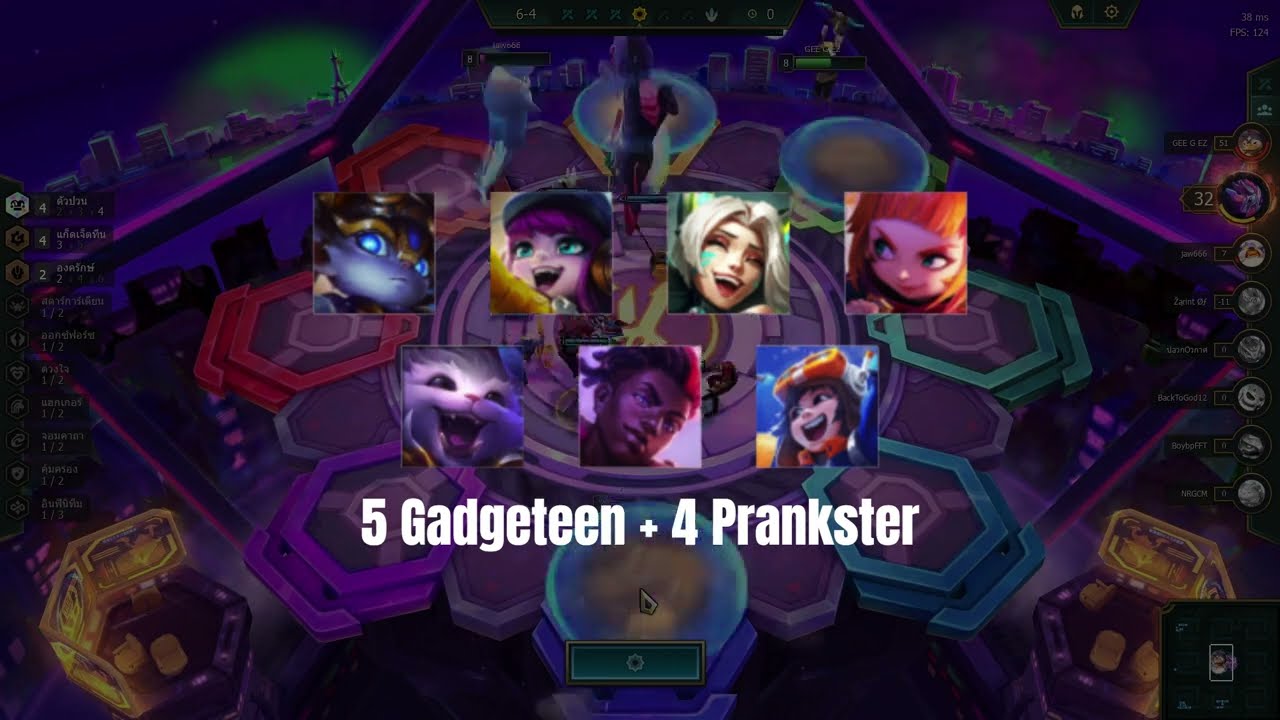The poster appears to be an advertisement or screenshot for a video game with a detailed, vibrant design set against a predominantly purple background. The main feature is a grid of seven avatars arranged in two rows—four on the top and three on the bottom. The top row features a diverse collection of characters: the first is a space creature that resembles a toddler with a pilot's hat and blue eyes, followed by three more human-like figures. The bottom row starts with a smiling cat in the first square, an African-American human in the second, and a cartoon girl in the third. Below these avatars, text in white reads "5 Gadgeteen plus 4 Prankster," indicating perhaps a split between two groups or categories within the game. The background of the poster is a complex mix of neon colors — purple, red, and aqua green — suggestive of a futuristic or space-themed cityscape, possibly resembling a spaceship or a pinball board. Dimly lit elements on the left and right sides display what appear to be player scores or usernames, hinting at this being a menu or results screen. Dark, faint characters can be seen on the right edge of the image, adding to the busy, intricate visual composition.